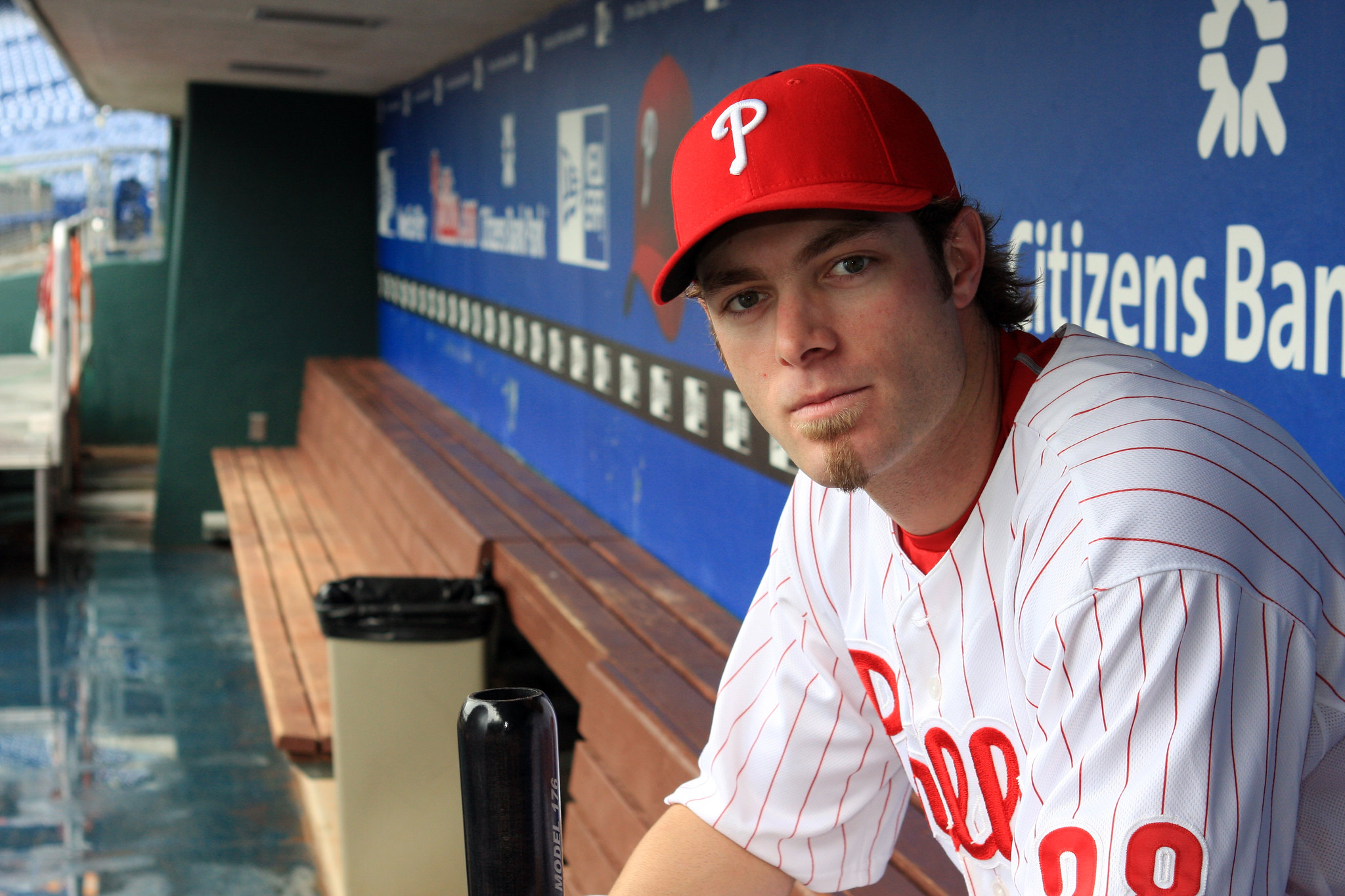This photograph features a Philadelphia Phillies player seated in the dugout, prominently positioned on the right side of the image. He is wearing a red cap emblazoned with a white "P" for Phillies and a white jersey adorned with red lettering that spells "Phillies." Red lines accent his jersey, and a partial view of his number, possibly 29 or 39, is visible on his arm. The player is holding the upper part of a bat in one hand. His expression is serious, and he sports a distinctive facial feature: a slight burn below his mouth along with a vertical strip of goatee that extends slightly across his chin.

The setting includes a blue wall with white text reading "Citizens Bank" behind him. He is seated on a brown wooden bench. Also in the background, there is a tan dustbin with a black liner to his left, contributing to the casual, candid atmosphere of the dugout scene.